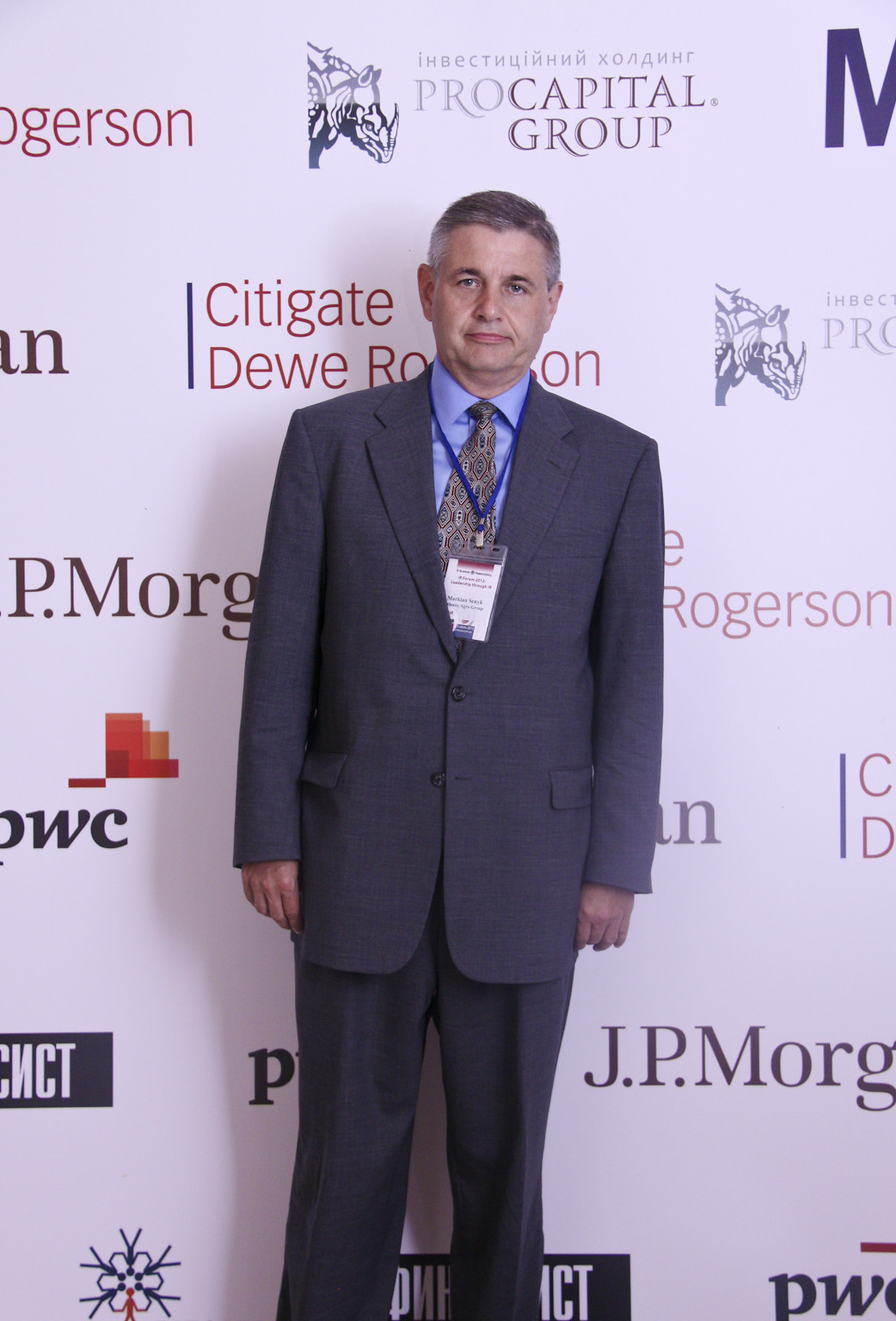In this detailed photograph, we see a middle-aged to older gentleman standing directly at the center, looking straight into the camera with a neutral expression. He is dressed in a well-tailored gray suit that matches his gray pants. Underneath the suit, he wears a blue dress shirt paired with a necktie featuring an intricate pattern of light brown, red, and perhaps some subtle tones of blue and black. Draped around his neck is a blue lanyard, suspending a plastic ID card that's not fully visible as it faces away from us.

The man’s hair is light brown in the middle with gray strands on the sides, and his face is marked with visible wrinkles, suggesting his older age. The setting is indoors, possibly at a corporate event, evident from the pristine white wall in the background that displays various brand names and sponsors. Prominently visible among them are Pro Capital Group at the top, followed by CityGate and J.P. Morgan among others. Some of the text appears clipped or partially obscured by the man’s presence. The overall appearance and detailed attire of the man, combined with the corporate logos, hints at a formal or professional gathering.